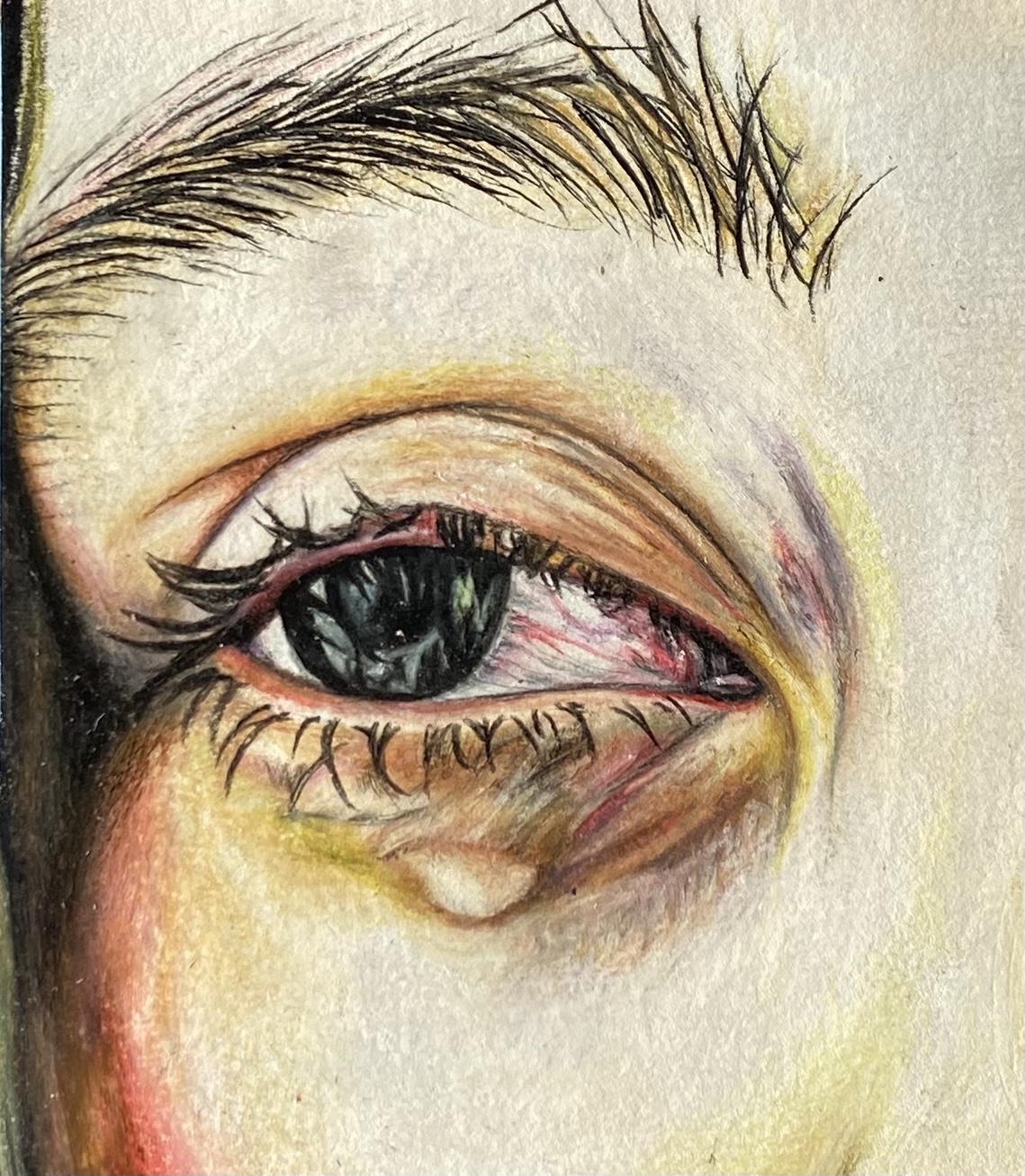This highly detailed, ultra-photorealistic colored pencil illustration focuses closely on a woman's right eye and eyebrow. She has pale, Caucasian skin with a noticeable bruise and dark discoloration beneath the eye. The eye itself is a striking dark green, but bloodshot, with visible red and purple veins in the corners. Her thick, dark black eyelashes accentuate the bloodshot effect. Her eyebrow, composed of intricately defined strands, features hairs that curve left and right, with some sticking straight up. The folds of her eyelids are meticulously drawn, adding to the realism. A tear is visible just below the lower eyelid, and there's some red discoloration on the cheek to the right. The woman appears to be gazing slightly to her right. Despite the close-up nature of the drawing, the intricacy of each element—from the individual hairs of the eyebrow to the veins in the eye—creates a compelling, almost lifelike portrayal of her emotion and physical state.